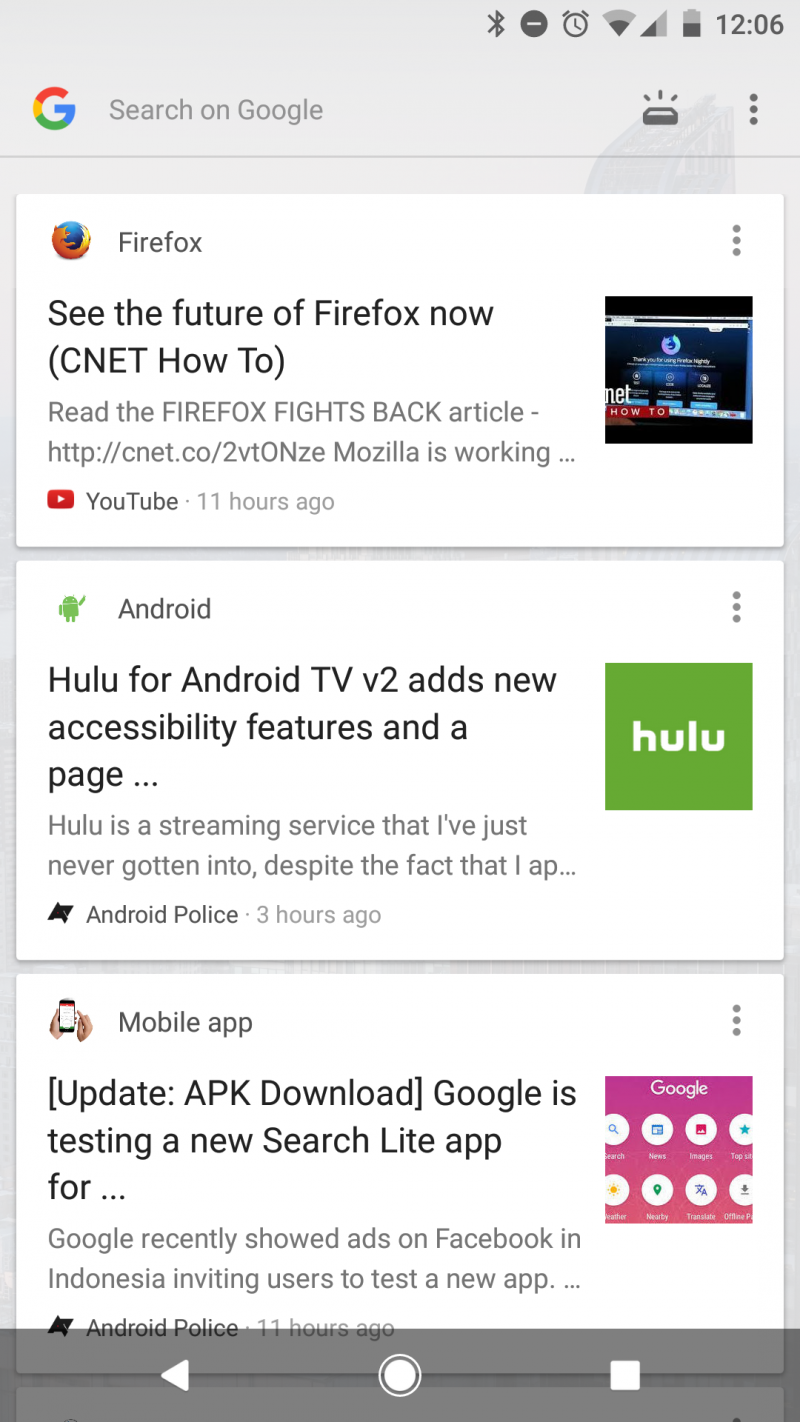The screenshot appears to be taken from a mobile device, likely an Android, displaying Google's news feed feature. At the top of the screen, the device's HUD shows essential status icons, such as the battery level, Wi-Fi connection, Bluetooth, and the clock, which reads 12:06. Beneath this, the recognizable Google logo and search bar occupy the top portion of the interface, allowing users to perform web searches directly.

Dominating the screen is Google's news feed, showcasing three distinct posts. The first post, sourced from Firefox, features a YouTube video. The second post, related to Android, is from the website Android Police. The third and final post at the bottom pertains to a mobile app, also shared by Android Police. These posts seem to highlight the topics of interest rather than the original source.

At the bottom of the screen, the device’s navigation buttons are visible, including the Back button, Home button, and the Overview button for managing open tabs.